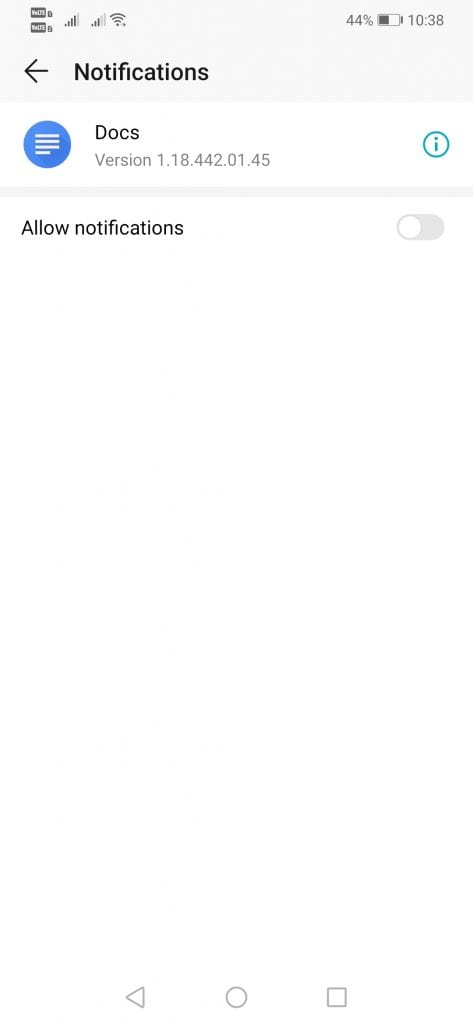The screenshot displays a cell phone at 10:38 AM, with a battery level of 44%. The device is connected to Wi-Fi and shows an active cellular signal. At the top of the screen, there is a back arrow next to the label "Notifications." The screen displays information about the "Docs" app, including the version number 1.1844.442.01.45, and features an information button represented by an 'i' within a circle. The option to "Allow notifications" is shown, and it is currently turned off. At the bottom of the screen, the navigation bar contains the standard icons: a back button, a home button, and a square button for toggling between open applications. The overall background is white, providing a clean and minimalistic look.